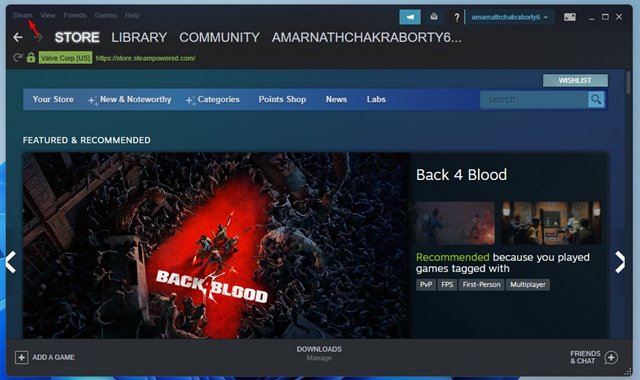The top portion of the interface displays a menu in all capital letters from left to right, reading: STORE (bolded, indicating it is likely selected), LIBRARY, COMMUNITY, and AMARNATH CHAKRABORTY... . Below this menu, on the left side, there is a grey refresh symbol followed by a mossy green lock icon. To the right of these icons, there is a green insignia with the black text "Valve Corp" followed by "(US)" in brackets. Adjacent to this is a URL bar with green text.

The background transitions from navy blue in the top left corner to a dark, almost grayish blue in the bottom right. At the bottom, there is another gradient menu, starting with a light navy blue on the left and transitioning to a deep royal blue on the right. The menu options are: YOUR STORE, NEW AND NOTEWORTHY (highlighted with sparkles on the left), CATEGORIES (also with sparkles), POINTS SHOP, NEWS, and LABS. To the right of these options is a teal-colored search bar, bordered in royal blue similar to the background. The search bar includes a magnifying glass icon set within a small light blue background box.

Below the search bar, the text "FEATURED & RECOMMENDED" is prominently displayed in capitalized white lettering. The primary image features a group of creatures watching another creature battling in an arena with a red floor. The title "BACK 4 BLOOD" is displayed in diagonal, blocky, distressed lettering, with the number "4" blending into the red background.